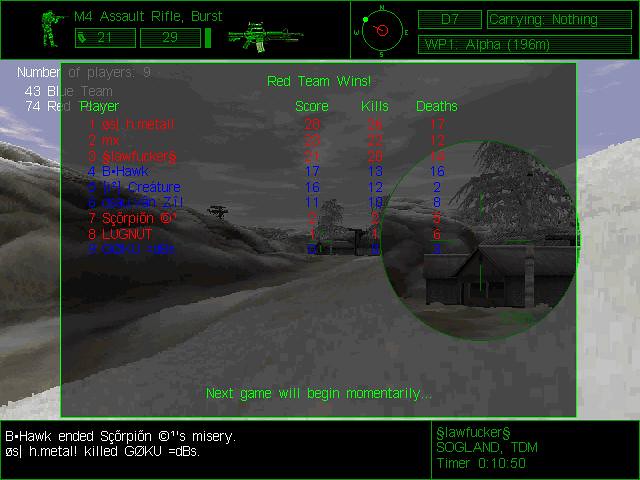A still image captured from a video game, framed with black banners displaying green text at the top and bottom. The gray-toned desert scene shows a barren road emerging from the left side and stretching into the vanishing point at the center. Towards the back, on the right side, an inset circle highlights a building resembling a longhouse, featuring two front-facing windows and no additional windows. A lone palm tree stands to the right of the building. In the top left corner of the image, a small character holding an M4 assault rifle is depicted, with the text "M4 Assault Rifle Burst" and numerical values displayed beneath. On the right side, a compass is shown alongside the text "D7 Carrying Nothing WP-1 Alpha 196 meters."